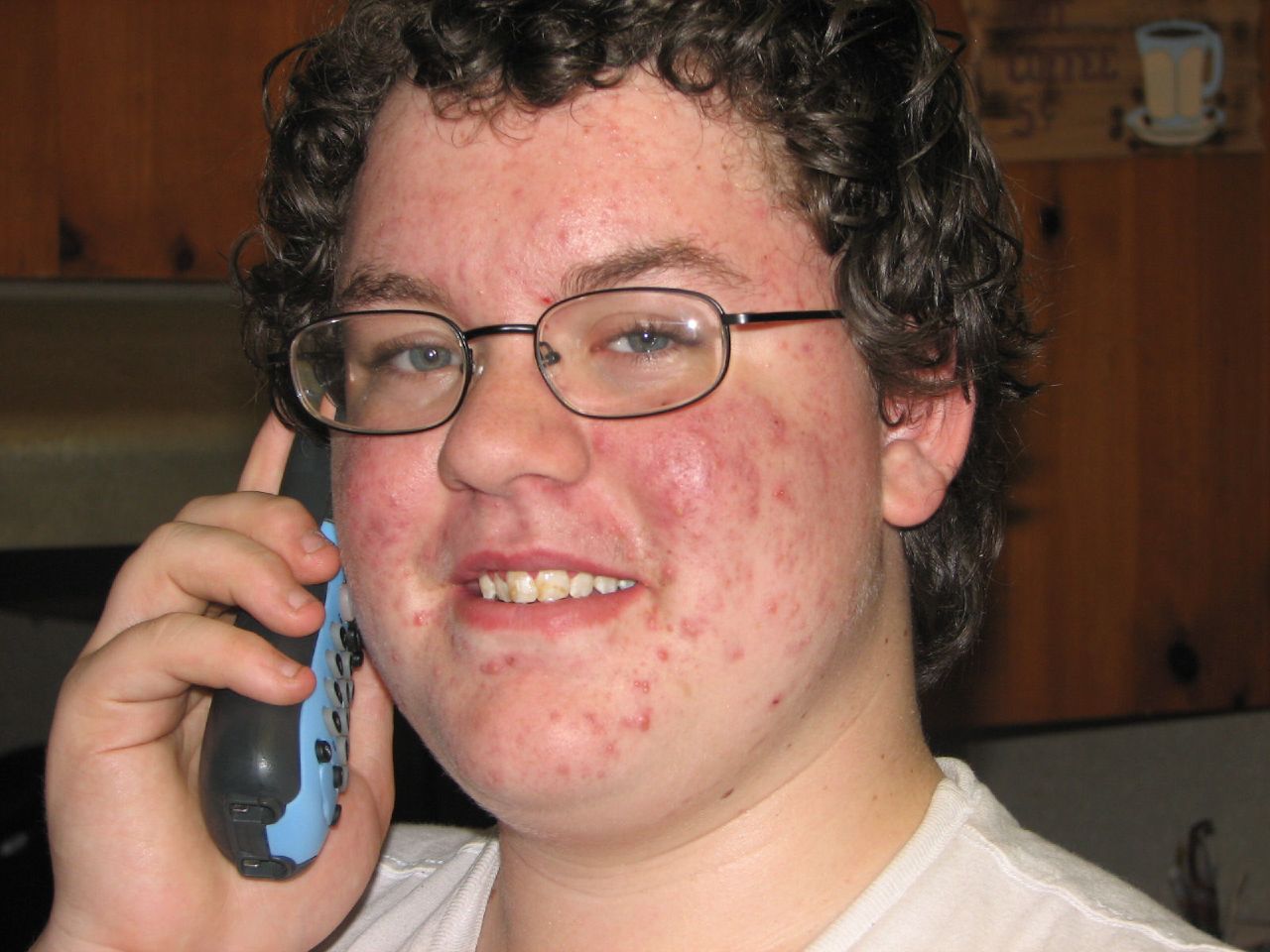This is a detailed full-color indoor photograph from the early 2000s or 2010s, featuring a close-up of a young man, likely in his early 20s. The primary focus is on his face, partly cropped at the top by the frame. He has a rounded, heavyset face with extensive acne and numerous freckles. His short, curly dark brown hair complements his blue eyes. He is wearing small, golden, dark-trimmed eyeglasses and a white T-shirt. The young man is smiling as he holds an old-style telephone with a black body and blue front, complete with white buttons, to his ear. His fingernails are noticeably bitten down to the quick, and he has a mole on his neck. Behind him, there are visible elements of a kitchen, including gray flooring, a black paneled wall, and wooden cabinets. In the upper right-hand corner of the image, a sign featuring a yellow mug with a white substance dripping down can be seen. Additionally, a white coffee mug and saucer rest on a browned counter in the background.